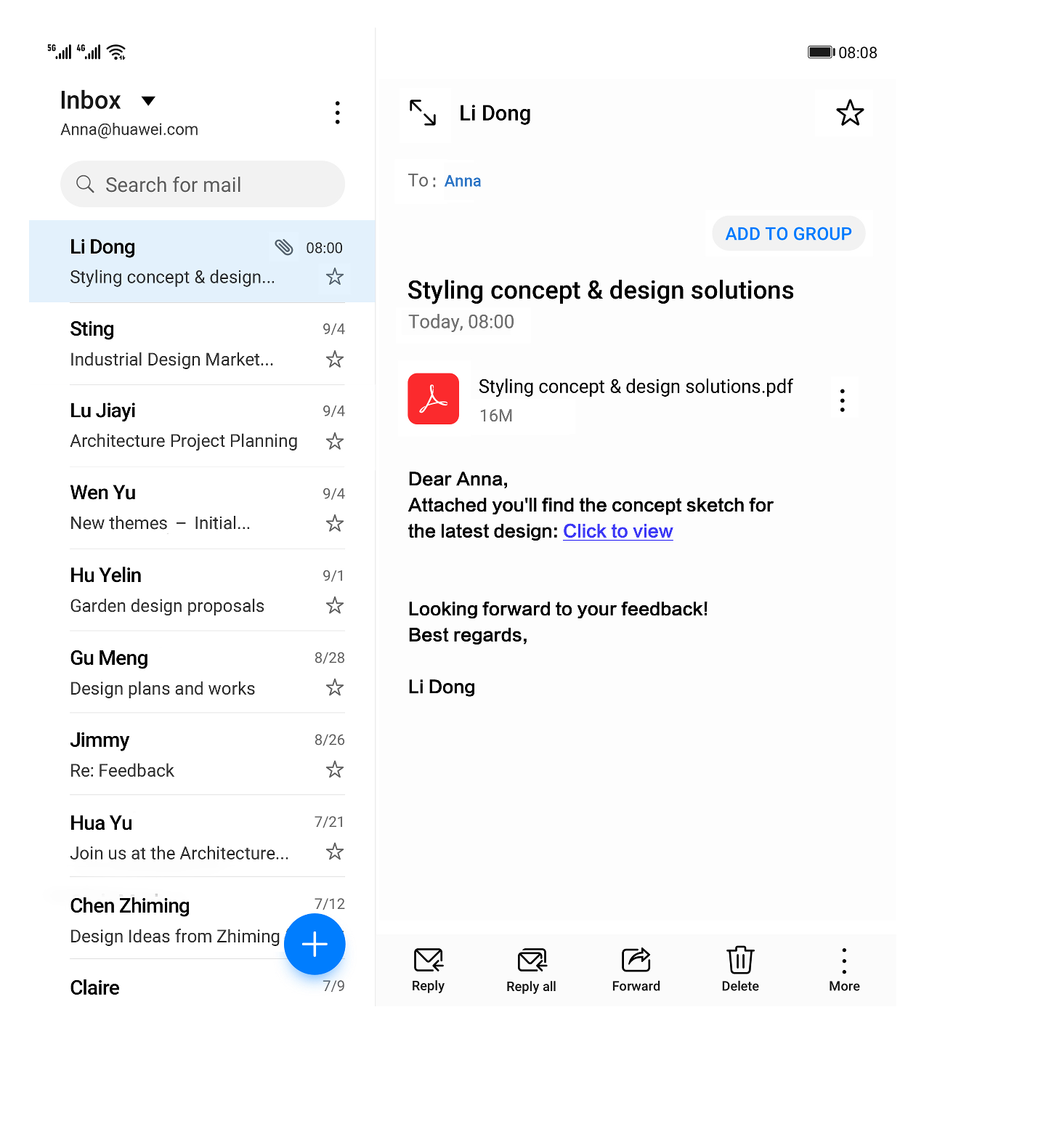This detailed and cleaned-up caption for the described image of an email inbox provides a thorough depiction:

---

The image displays an email inbox interface. In the top-left corner, the word "Inbox" is prominently displayed with an arrow pointing downwards. Below it, there is an email address: "Anna@Huawei.com." Adjacent to this, there is a search bar labeled "Search for mail" accompanied by a magnifying glass icon.

The list of senders includes names like Li Dong, Sting, Lu Jie, Wen Yu, Hu Yelin, Guo Ming, Jimmy, Hua Yu, Chen Zhaoming, and Claire. On the right side of the interface, an open email from Li Dong is visible. The email is addressed to Anna, featuring a blue hyperlink labeled "Add to group." The subject line reads "Styling Concept and Design Solutions," dated today at 8:08.

Attached to this email is a PDF titled "Styling Concept and Design Solutions," sporting an Adobe Acrobat logo and a file size of 16 megabytes. The email body begins with "Dear Anna," followed by a message indicating: "Attached you'll find the concept sketch for the latest design," with "click to view" available as a blue hyperlink. The email concludes with "Looking forward to your feedback. Best regards, Li Dong."

At the bottom of the email, there are several action buttons. These include "Reply" (an envelope icon with an arrow pointing left), "Reply All" (multiple envelopes), "Forward" (a box with an arrow pointing right), and "Delete" (a trash can icon). There are also three dots indicating additional options under the "More" button. In the top-right corner, the current time is displayed as 8:08.